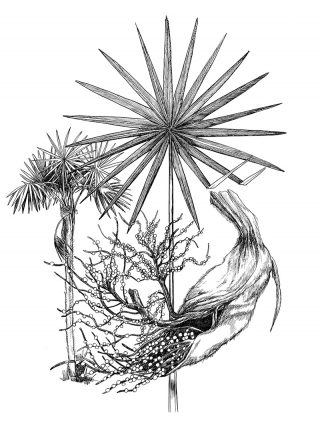This black-and-white botanical illustration on a plain white background depicts a meticulously detailed plant, possibly resembling a palm tree, drawn with pencil or charcoal. At the top of the tall, thin stalk is a star-like arrangement of slender, pointy leaves, numbering around fourteen or more, radiating outward. The bottom right features an intriguing, conical-shaped root or seed pod, partially opened to reveal smaller extensions that resemble miniature trees adorned with tiny white dots, which might be seed beads. The intricate shading and fine detailing bring a sense of depth and realism to the abstract, artsy depiction of the plant's complex structures.